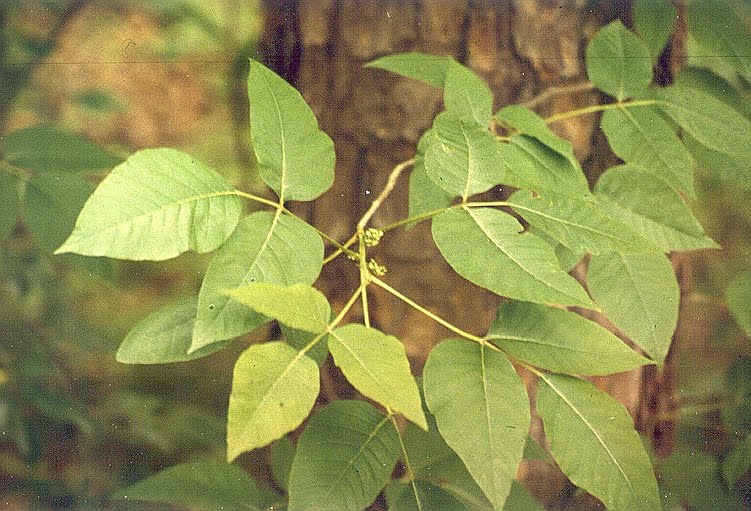The photograph captures a close-up of green leaves in front of the trunk of a tree, which is slightly offset to the right. The tree trunk is broad and displays a brown, bark-textured surface. Surrounding the trunk and filling much of the image are leaves in various shades of green. Most of the leaves are a neutral or dull green, with some appearing darker and slightly blurry in the background. Toward the front center of the image, between two clusters of dark green leaves, a trio of light green leaves emerges distinctly from a stem. The background beyond the tree trunk, although blurred and somewhat obscured, suggests the presence of more leaves and a small area of light brown, possibly dirt, adding to the natural outdoor setting. The overall composition emphasizes the greenery and the interplay of light and shadow among the leaves.